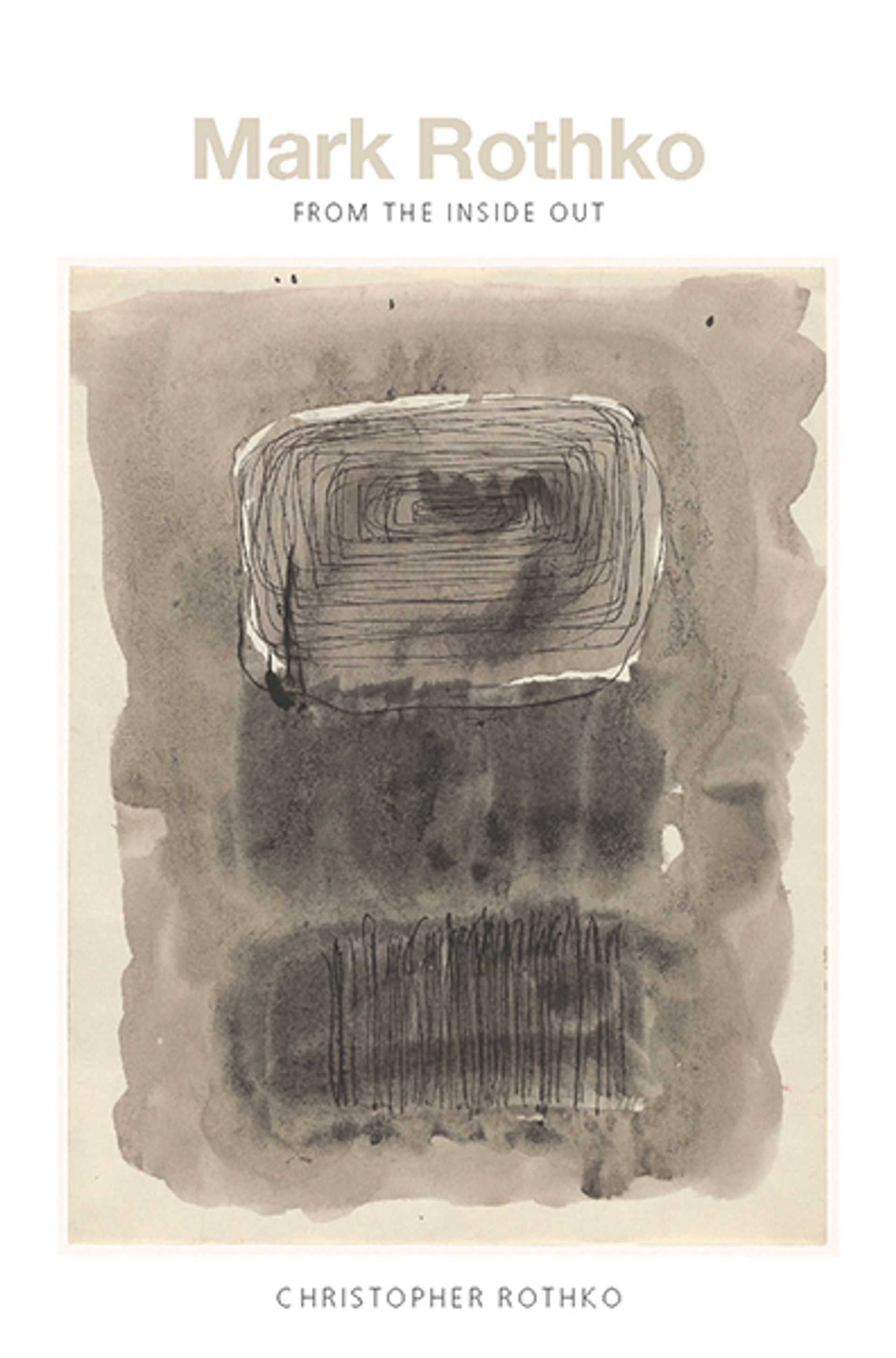This is an image that appears to be the cover of a book titled "From the Inside Out" featuring the work of Mark Rothko. The design is visually striking with a mix of colors and text layout. At the top, the name Mark Rothko is displayed in a light beige color, distinctively not in all capital letters, and possibly in an Arial font. Below this, the book title "From the Inside Out" is written in a dark gray font, which matches the font used for Christopher Rothko's name at the bottom, both in all capital letters. The central artwork showcases a washed-out, watercolor-like painting in dark gray tones. The piece has a rectangle form with black marks and somewhat spiral shapes within a square, adding a dynamic visual element. The overall background remains white, allowing the dark and tan hues in the artwork to stand out clearly, resulting in a sophisticated and textured appearance.